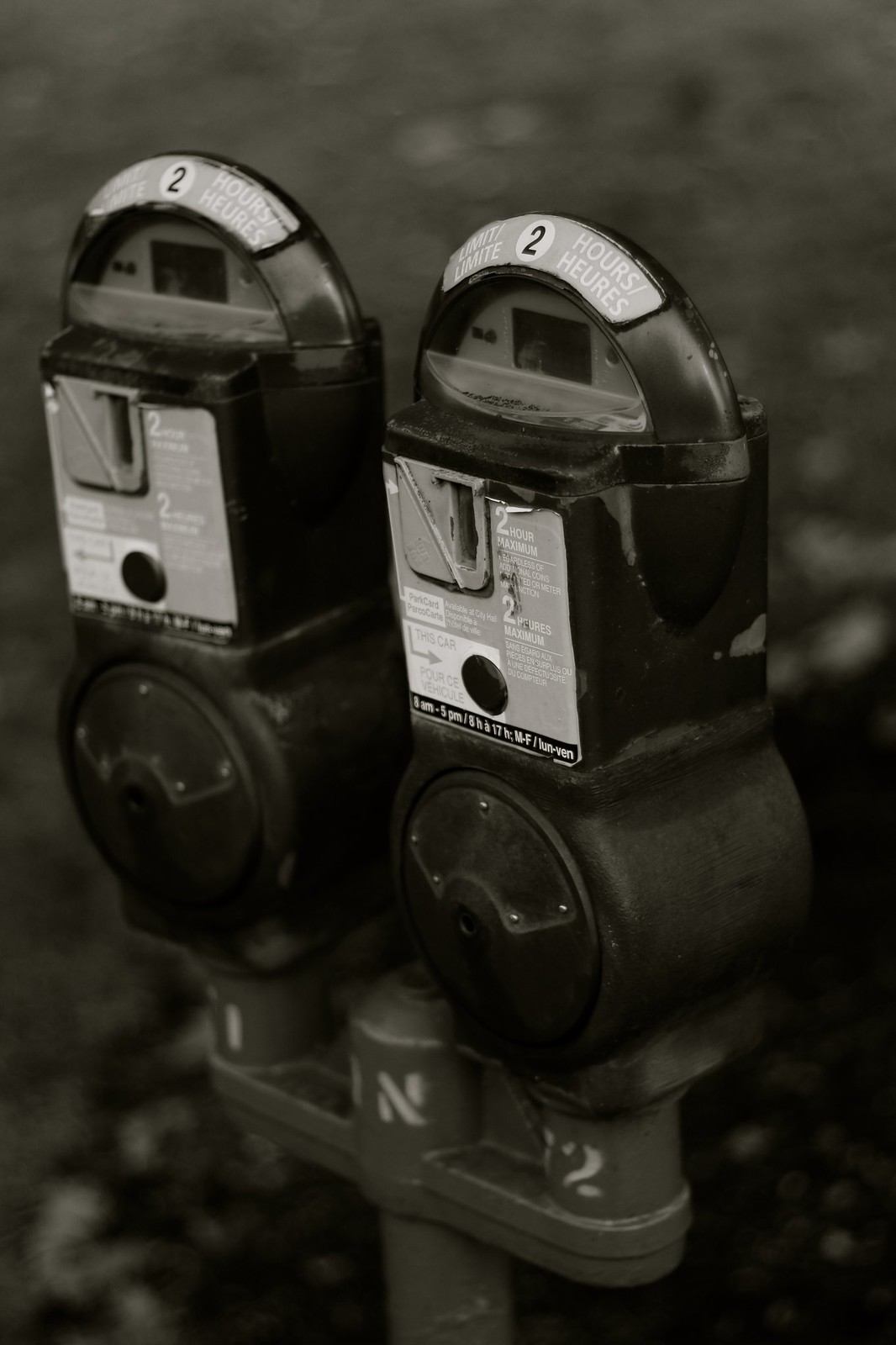The image is a black-and-white photograph taken outdoors, centered on a pair of vintage parking meters mounted on a single pole. The background is blurred, highlighting the meters and giving the photo an artistic feel. Both meters, which appear old-fashioned and worn with paint chipping off, are identical and prominently display the number "2" on their curved tops, indicating a two-hour maximum parking limit. The information is presented in both English and French, with labels such as "hours, heures" and a note stating "2-hour maximum" from 8 a.m. to 5 p.m. Each meter features a small rectangular glass window, a coin slot, and a large circular metal section at the bottom. The pole, resembling a trident with three prongs, has numbers "11" and "12" inscribed on it. The photograph’s sharp focus on the meters against the blurred background enhances the detailed textures and elements of the meters, from the metal bases to the blackened circular rivets at the bottom.